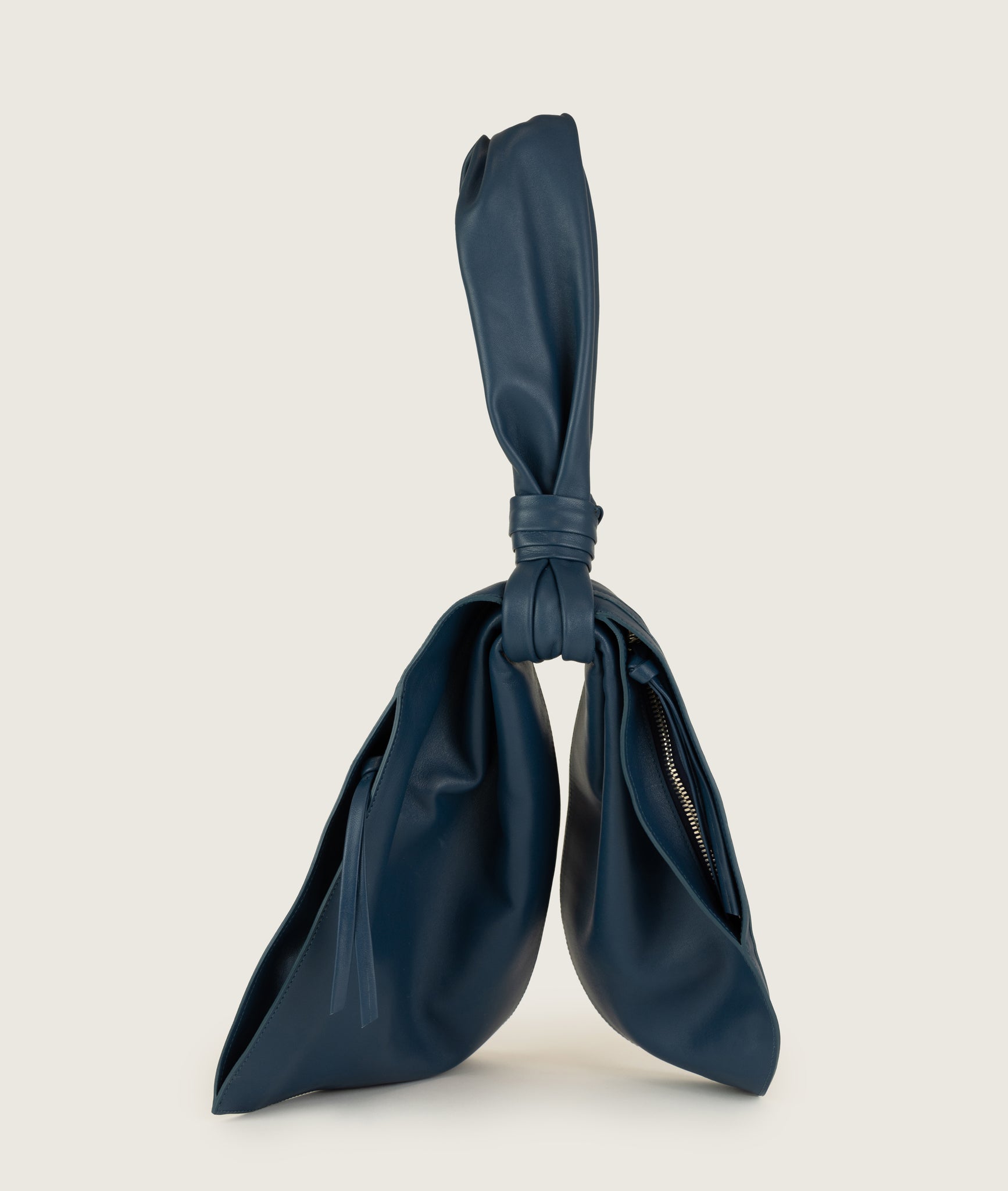The image depicts a vertical rectangular composition with a primarily white background. Central to the image is an intricately arranged black scarf, made of a soft and textured material, reminiscent of velour. The scarf is tied at its midpoint, giving the impression of two legs hanging down. Interlaced with this black scarf is another scarf, also seemingly heavy, which is tied around the middle section of the first scarf. The ends of this second scarf are sticking straight up, creating a peculiar and visually striking configuration. Notably, the black scarf features a small mark along one of its sides. Despite initial impressions that it might resemble a tie or a purse, the unusual arrangement and zipper detail on the folds suggest a more complex and possibly artistic display of the scarves.